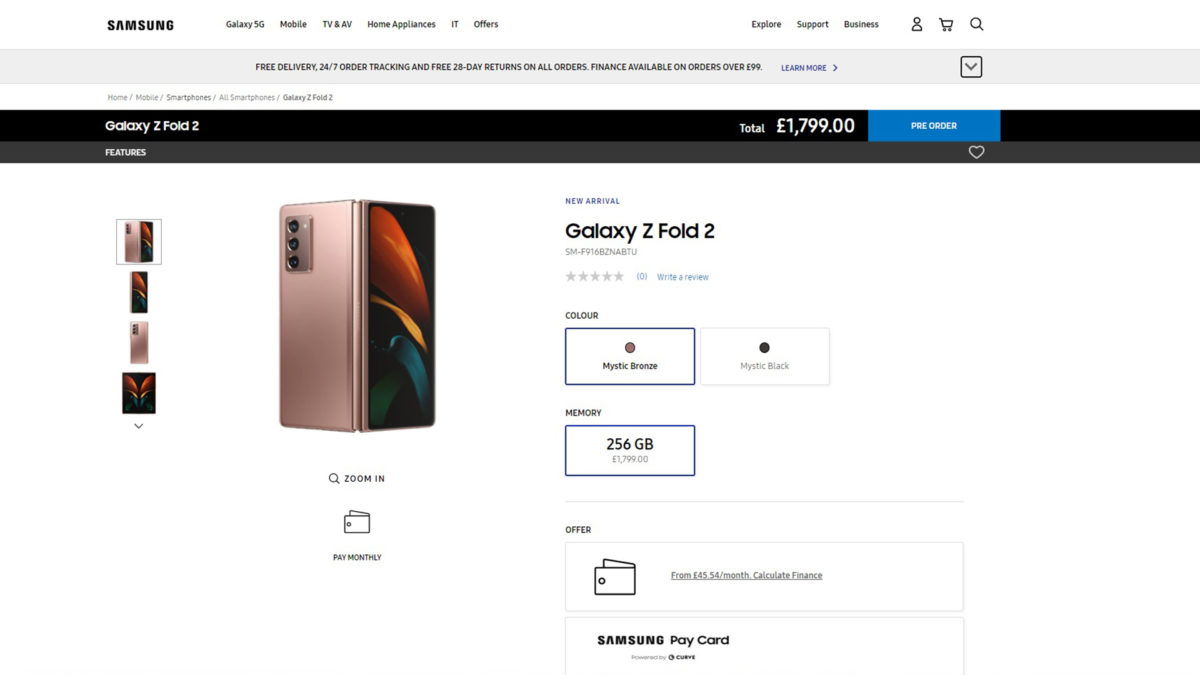In the upper left corner of the image, the word "Samsung" is prominently displayed in bold, black, capital letters. To the right of this, the navigation options are listed as "Galaxy 5G," "Mobile," "TV & AV," "Home Appliances," and "Offers." Approximately four inches further to the right, there are additional navigation links: "Explore," "Support," and "Business," all in black text.

Beneath this section, a long gray bar spans the width of the image, featuring promotions that read: "Free Delivery 24/7," "Order Tracking," and "Free 28-Day Returns on all orders." It also highlights that "Finance available on orders over $99."

Below the gray bar, a long black bar appears with the product details. To the left, it reads "Galaxy Z Fold 2" followed by the price "$1,799.00" in smaller text. A blue box next to this text indicates that the item is available for "Pre-Order."

Directly below the black bar is an image of the Galaxy Z Fold 2 phone, showcased in a stunning rose gold color with three camera lenses visible. To the right of the phone image, the product name "Galaxy Z Fold 2" is displayed. Above this, the label "New Arrival" is printed, and the available colors are noted as "Mystic Bronze" or "Mystic Gray." Just below, the memory specification "256 GB" is provided. At the very bottom of the image, "Samsung Paycard" is mentioned in black text.